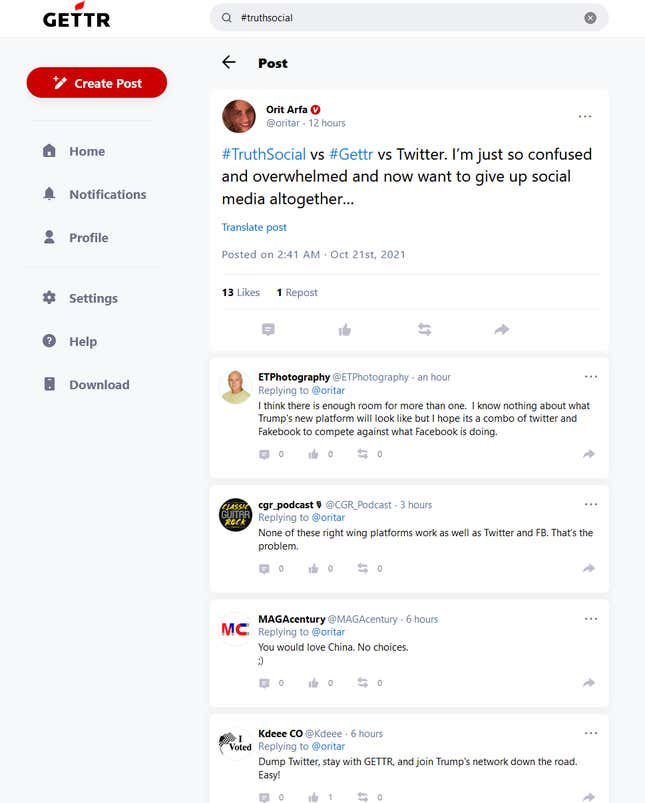The image depicts the homepage of the social media platform GETTR. The screen displays the GETTR logo prominently at the top, alongside a conspicuous red button labeled "Create Post." Just below the header is a horizontal menu bar with six tabs: Home, Notifications, Profile, Settings, Help, and Download.

In the main section of the page, user Orit Alpha has posted a message: "Hashtag truth social versus hashtag Getter versus Twitter. I'm just so confused and overwhelmed I now want to give up social media altogether."

Below this post, there are four responses from other users:
1. ET Photography: "I think there is enough room for more than one. I know nothing about what Trump's new platform will look like but I hope it's a combo of Twitter and Facebook to compete against what Facebook is doing."
2. CGR Podcast: "None of these right-wing platforms work as well as Twitter and Facebook. That's the problem."
3. A third user has made a sharp remark: "You would love China, full stop, no choices."

The image captures the dynamic and sometimes contentious nature of discussions on social media platforms.